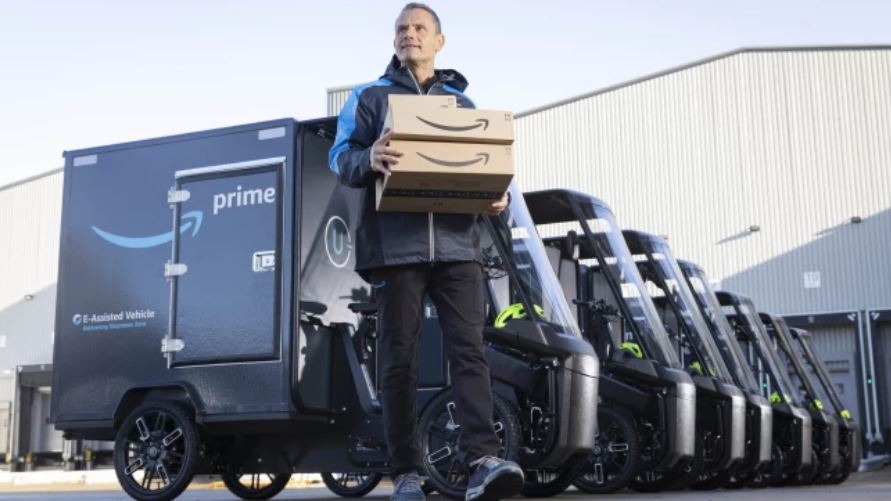A daytime photograph captures an Amazon delivery worker in the middle of an outdoor commercial complex filled with activity. The image prominently features a blue sky occupying the upper left and top sections of the frame, providing a clear and crisp backdrop. The delivery person, a Caucasian man in his 40s or 50s, is mid-stride while carrying three Amazon boxes, suggesting he's in the midst of his delivery duties. He is dressed in black pants, sneakers, and a distinctive Amazon blue jacket with a hood.

The background showcases a large warehouse with light-colored siding and several truck docking stations clearly visible, indicating a bustling logistics hub. Directly behind the delivery worker is a perfectly aligned row of seven electric, three-wheeled delivery vehicles, each adorned with the recognizable Amazon smile logo and the word "Prime." The cargo boxes on these vehicles also feature the words "e-assisted vehicle," highlighting Amazon's commitment to eco-friendly delivery solutions. The overall scene combines elements of modern logistics, sustainability, and a focused human effort in the fast-paced world of e-commerce.